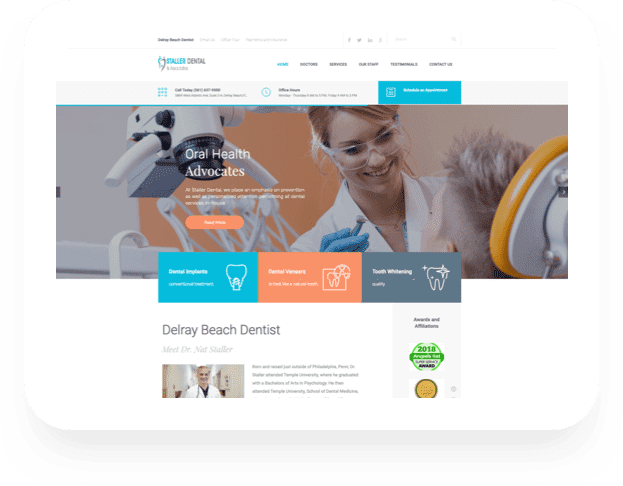**Description:**

The image appears to be a low-resolution screenshot from a dental clinic's website, predominantly featuring a white background. At the top of the image, the clinic's name, "Staller Dental," is displayed, with "Staller" in light blue text and "Dental" in dark gray, accompanied by a tooth icon that matches the color scheme (half blue, half dark gray). To the right of the clinic's name, several clickable links are listed: Home, Doctor of Services, Our Staff, Testimonials, and Contact Us.

Below the header, there is a large banner image spanning the width of the screenshot. This banner showcases a female dentist—a young, blonde woman wearing safety glasses—smiling and looking down at a patient whose face isn't fully visible. The patient has short, blonde hair. In the background, various dental or medical equipment is visible, emphasizing the clinical setting.

Further down, the image is divided into three colored segments, each promoting a specific dental service: "Dental Implants" in blue, "Dental Veneers" in orange, and "Tooth Whitening" in gray. Beneath these segments, text reads "Delray Beach Dentist, meet Dr. Nat Staller," accompanied by a photograph of Dr. Nat Staller.